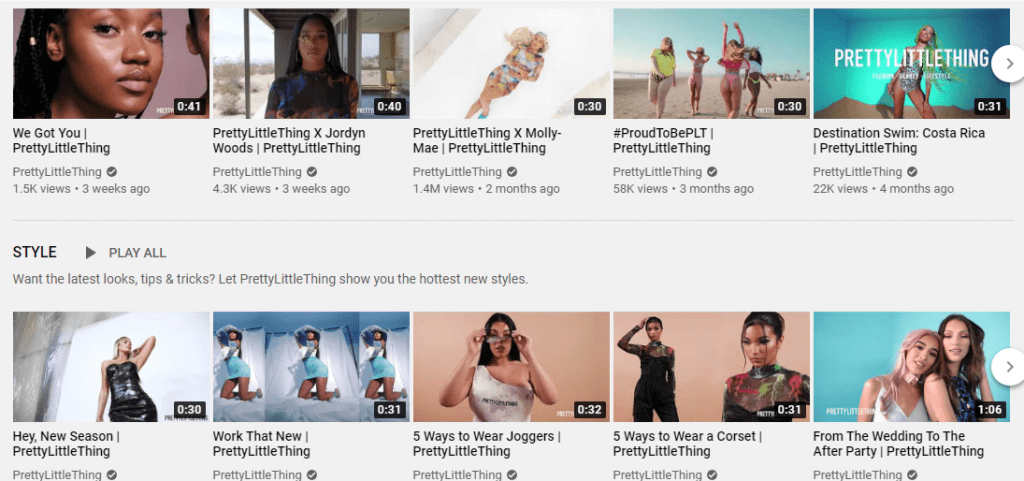The image depicts a YouTube page showcasing a selection of short videos. The videos are arranged in two horizontal rows, each featuring content from the channel "PrettyLittleThing" (notably formatted as one continuous word). The videos have varying lengths, mostly between 30 to 40 seconds, with the longest being 1 minute and 6 seconds.

In the first row, the videos from left to right are titled: "We Got You," "PrettyLittleThing x Jordyn Woods," "PrettyLittleThing x Molly Mae," "Proud to be PLT," and "Destination Swim: Costa Rica." Each video is presented with a unique thumbnail image.

The second row of videos includes the titles: "Hey New Season," "Work That New," "Five Ways to Wear Joggers," "Five Ways to Wear a Corset," and "From the Wedding to the After Party." The thumbnail for the final video in this row intriguing shows two women snuggled together, suggesting a romantic connection.